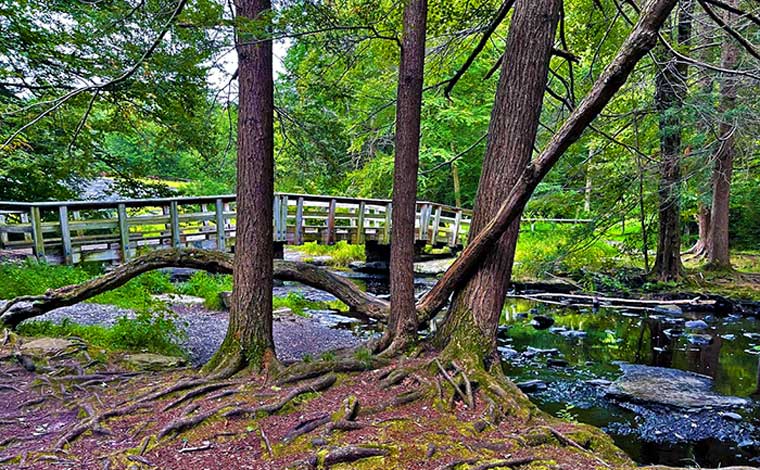This photo captures a serene natural scene, likely taken in a park or forested wetland area. At the forefront, there are three straight cedar trees with above-ground roots, accented by green moss at their bases. A fourth tree grows horizontally at the base of these three before rising vertically. A large fallen branch is wedged among the trees. The ground is a mix of brownish-yellow earth with small patches of gravel, and signs of sunshine peek through the canopy above and illuminate the area. A simple white wooden bridge with metal railings spans a narrow, dark stream or bog. To the right, some debris floats in the water, adding to the wetland atmosphere. The background features a dense, green forest, with additional conifer trees and leafy branches reaching towards the sky, which is partly visible with patches of clouds. The scene is tranquil, suggesting the peacefulness often found in nature.